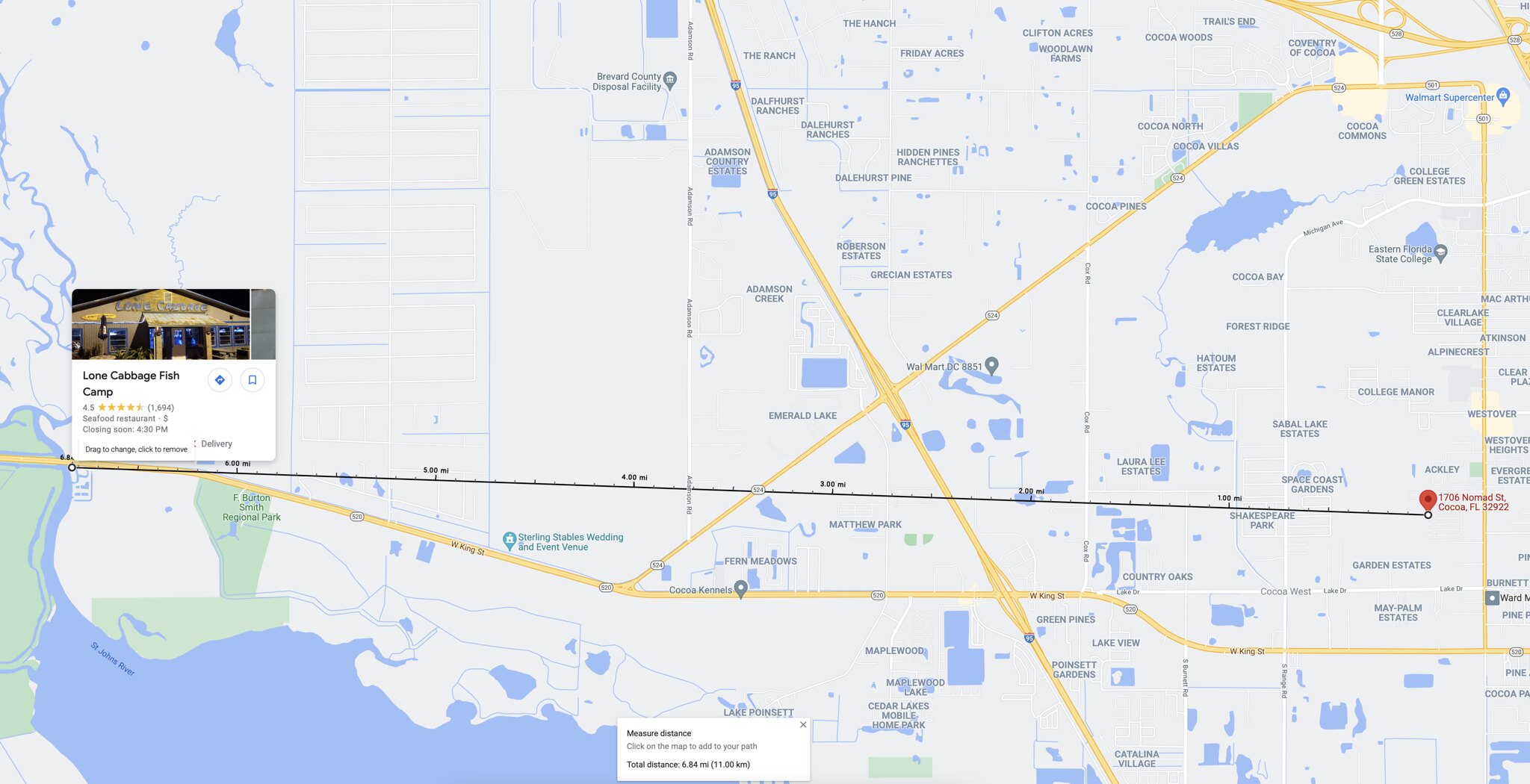This detailed map showcases a specific route in Florida. The route is marked by a straight line that extends from one end of the map to the other. On one end, there is a marked building referred to as either the "Lone Cabbage" or "Lone Carriage," though the precise name is not legible. There's an illustration of this building to aid in identification. At the other end of the route, there's another location, also marked, with an unreadable address. The map features a bluish-gray background with dark blue areas indicating bodies of water. Along the route, there are several markers denoting measurements at regular intervals, though the exact distances and additional annotations on the map are difficult to decipher due to the small size of the letters.